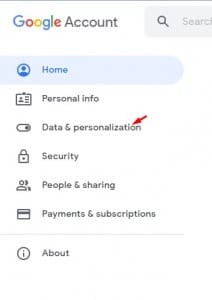A detailed descriptive caption for the image could be:

"The image depicts a screenshot of a Google Account settings page. At the top, the recognizable Google logo is prominently displayed, with a partially visible search box situated on the right-hand side—its 'search' text truncated due to the cut-off edge of the screen. The 'Home' tab is highlighted, indicating the current section being viewed. Adjacent to it is an empty, default profile picture icon. Below 'Home', a vertical list of menu options is visible, starting with 'Personal Information'. The 'Data & Personalization' section is emphasized with a small red arrow, suggesting a point of interest or required action within that tab. Following this, the menu continues with 'Security', 'People & Sharing', 'Payments & Subscriptions', and concludes with 'About' at the bottom. The emphasis on the 'Data & Personalization' section hints that it may be the destination for customizing settings, potentially related to changing the background or profile picture."